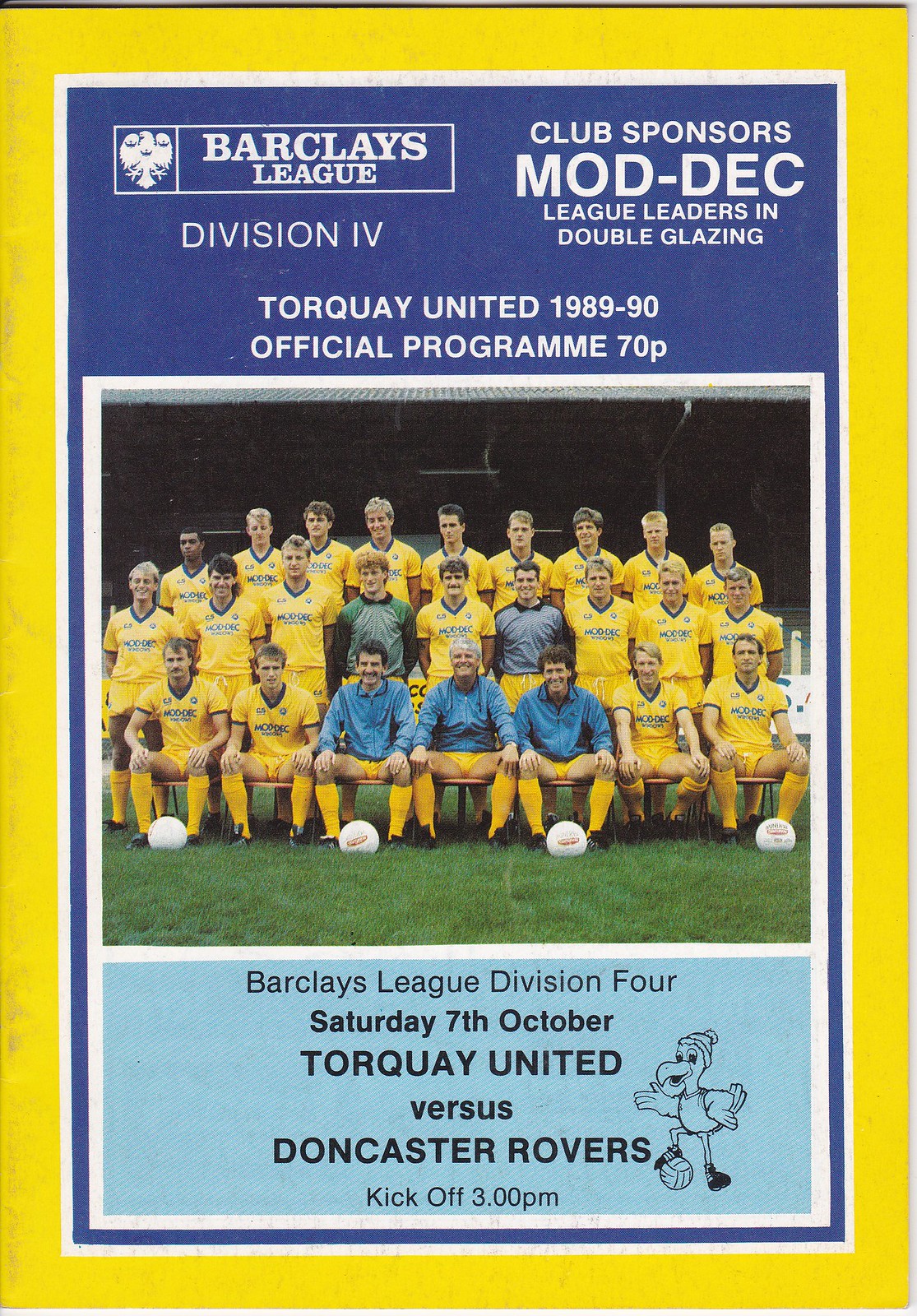The cover of the soccer program features a vibrant and detailed design centered around a team photo. The program, from the 1989-1990 season of the Barclays League Division 4, prominently highlights a match between Torquay United and Doncaster Rovers, taking place on Saturday, 7th October, with a kickoff at 3 p.m. The background of the cover incorporates a yellow border and segments of dark and light blue. In the top left corner, the white text reads "Barclays League" accompanied by its logo. On the top right, more white text indicates "Club Sponsors Mod-Dec League Leaders in Double Glazing."

The main image features the Torquay United team posing in their mostly yellow uniforms. Three team members in the front row wear blue jackets, possibly goalies, while additional figures in the back row sport dark jerseys, likely coaches. Four soccer balls are positioned on the grass in front of the team. The bottom section of the program, against a light blue background, reiterates the match details in black print, with a small cartoon drawing of a duck kicking a soccer ball to the right of "Doncaster Rovers." The official program price, "70 pence," is also noted near the top. The overall setting of the image is well-lit by natural light, making the colors and details clear and vivid.